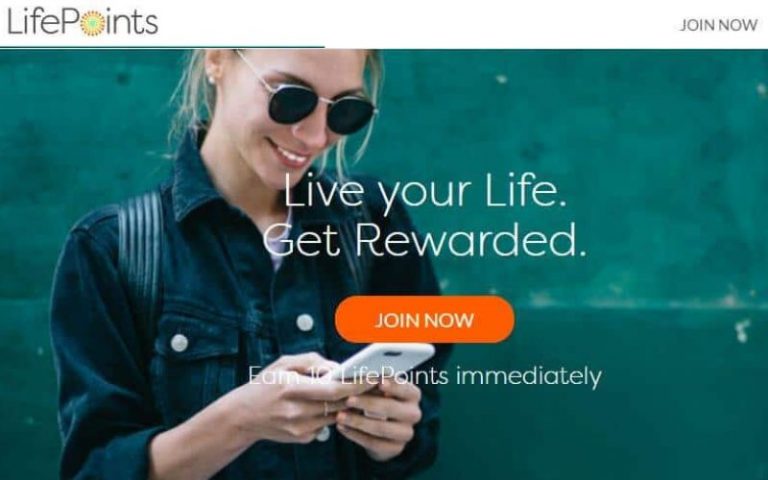In this vibrant and engaging webpage image, a smiling woman is seen wearing sunglasses and a stylish jacket while holding a white mobile device. Her expression suggests she is enjoying her experience on the device. Located at the top right corner is a call-to-action button labeled "Join Now." The prominent caption on this image reads, "Live your life, get rewarded. Join now, earn 10 Life Points immediately," inviting users to sign up and start earning rewards. The image features a color palette of green, blue, black, and white, creating a modern and appealing aesthetic.